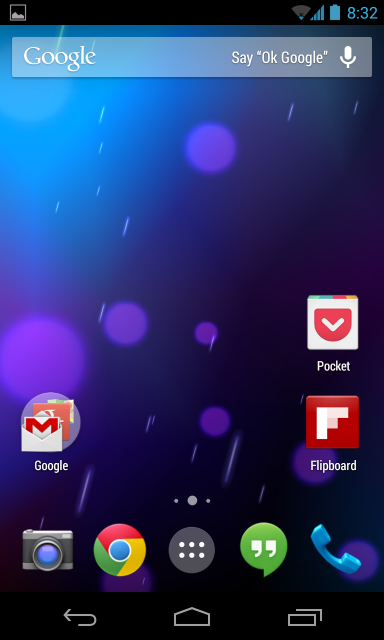A detailed, cleaned-up caption for the image could be:

"This portrait-oriented color screenshot captures the home screen of a mobile phone. At the top of the screen, the Google search bar is prominently displayed alongside the option to activate voice search with 'Okay, Google'. The status bar shows the time as 8:32, with full battery life and strong cellular reception indicated by four bars. The phone’s background features an abstract design with a gradient from dark to light blue, accented by streaks of light and bubble motifs. The home screen layout is minimalist, with visible app icons including Pocket, Flipboard, and Google placed sparingly towards the top. At the bottom of the screen, a dock houses the essential apps—Camera, Chrome, Text, and Phone—that remain consistent across all home screen pages. The navigation bar at the very bottom offers buttons for going back, returning to the homepage, and viewing multiple open windows."